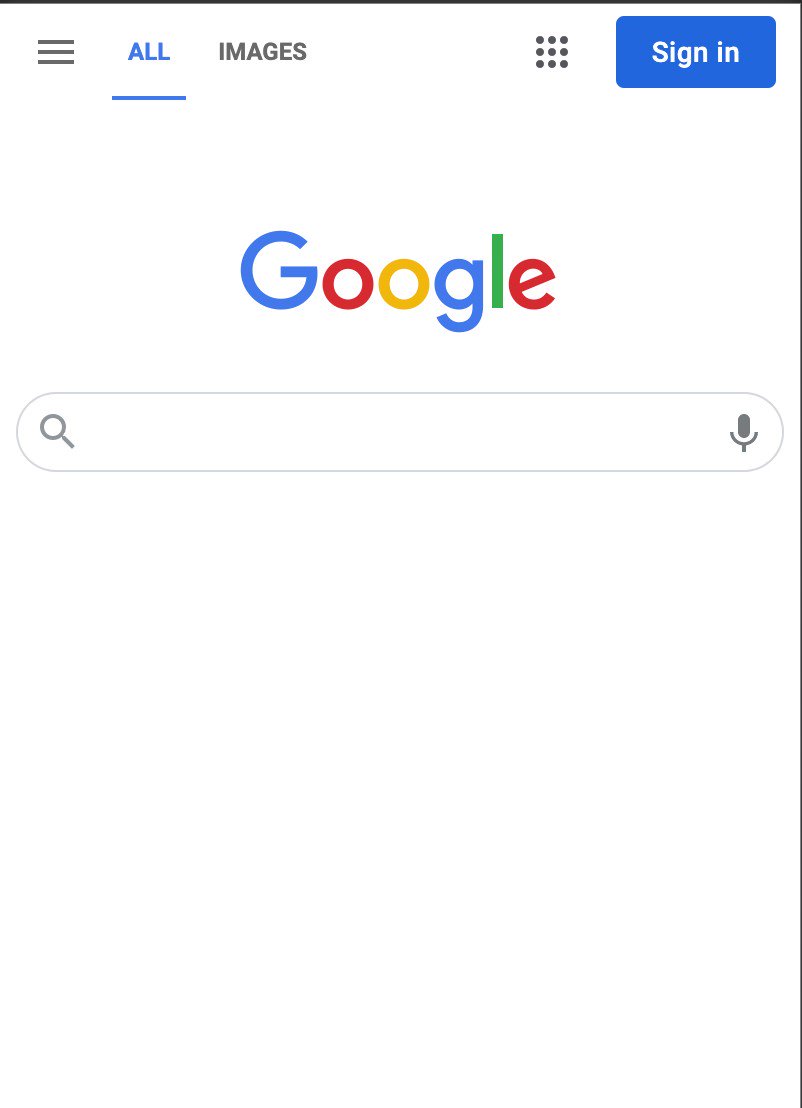This is a detailed screenshot of the Google homepage. At the top-left corner, there are three horizontal bars that can be clicked to open the menu. Next to this button is the word "ALL," displayed in blue and underlined, indicating it is the current selection. Next to "ALL" is the word "IMAGES," written in uppercase grey letters. On the far right, there is a square icon composed of nine grey dots, which typically opens additional Google apps. Adjacent to this is a blue "SIGN IN" button with white text.

The majority of the page is a clean white background. Centered prominently is the Google logo, showcasing a capital 'G' in blue, followed by lowercase letters 'o' in red, 'o' in yellow, 'g' in blue, 'l' in green, and 'e' in red, all in a sans-serif font. Below the logo is a search bar that spans roughly the width of the screen. To the left of the search bar is a magnifying glass icon, signifying the primary search function, while to the right, there is a microphone icon, indicating the option for voice searches.